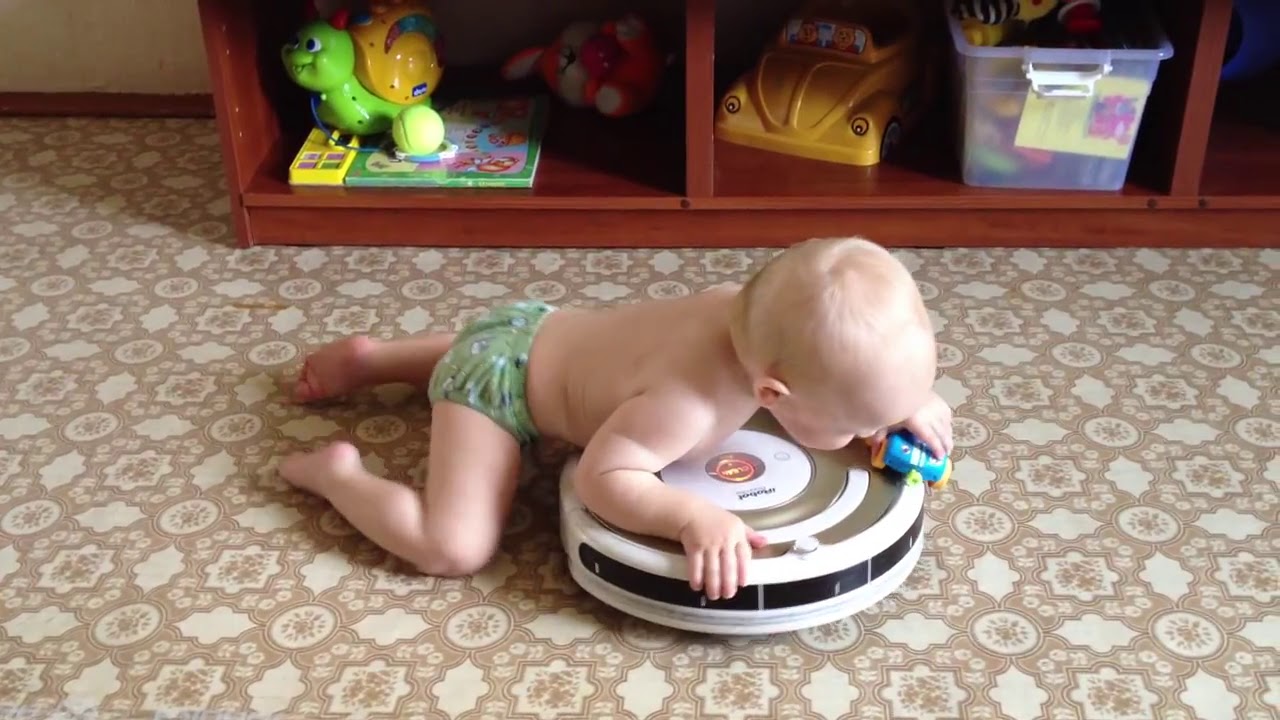In this indoor photograph, a Caucasian, blonde-haired baby—approximately six to nine months old—is lying with his legs sprawled out and arms hugging a modern, circular floor vacuum, likely a Roomba. The baby, who appears to be wearing a green diaper and no other clothing, has a blue toy car in his left hand. He is positioned slightly towards the bottom but mostly in the center of the image, on a floor that appears to be either linoleum or very closely cropped Raven carpet tiles with a dusty rose color and white rounded geometrical designs. Behind the baby, there is a stained wooden shelving unit with multiple cubbies. The left cubby holds a green plastic dragon, a box of crayons, a ball, and a children's book featuring buttons for interactive stories or sounds. The right cubby contains a yellow car and a purple plastic bin filled with toys. The background wall is white, accented with a brown baseboard. The overall setting and style of the Roomba suggest the photo was taken within the last decade.